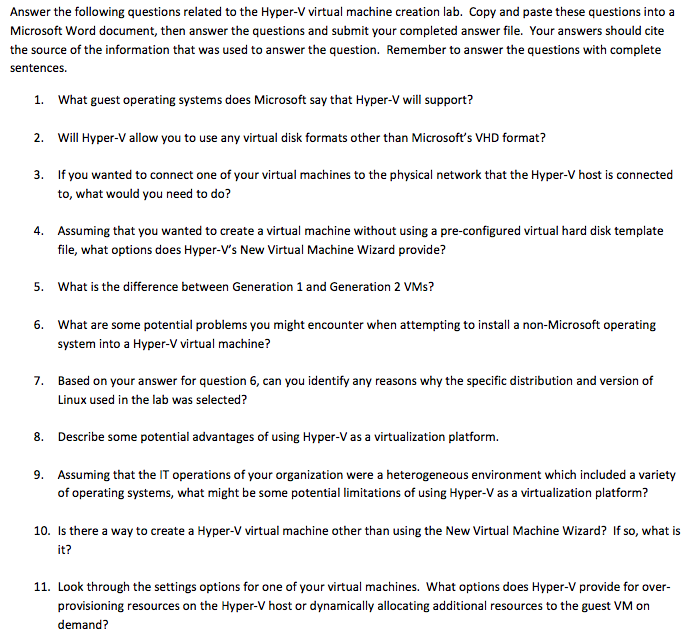The website depicted in the black and white image provides a detailed instructional guide for completing a Hyper-V virtual machine creation lab. At the top, the page prompts users to "Answer the following questions related to the Hyper-V virtual machine creation lab." It instructs users to copy and paste a list of questions into a Microsoft Word document, answer them, and submit the completed file. It emphasizes that answers should be in complete sentences and should cite sources used for information.

The eleven questions listed on the website cover various aspects of working with Hyper-V virtual machines. For instance, question one asks which guest operating systems are supported by Hyper-V according to Microsoft. Another question probes whether Hyper-V allows the use of virtual disk formats other than Microsoft’s VHD format. Additional questions inquire about network connectivity for virtual machines, options available in Hyper-V’s new virtual machine wizard for creating VMs without a pre-configured virtual hard disk template, and the differences between generation 1 and generation 2 VMs. Other questions explore potential issues when installing non-Microsoft operating systems and discuss the advantages of using Hyper-V.

Finally, the page directs users to review the settings options for one of their virtual machines, suggesting a final hands-on activity to tie the concepts together. This website serves as a comprehensive resource for anyone learning to navigate and manage Hyper-V virtual machines efficiently.